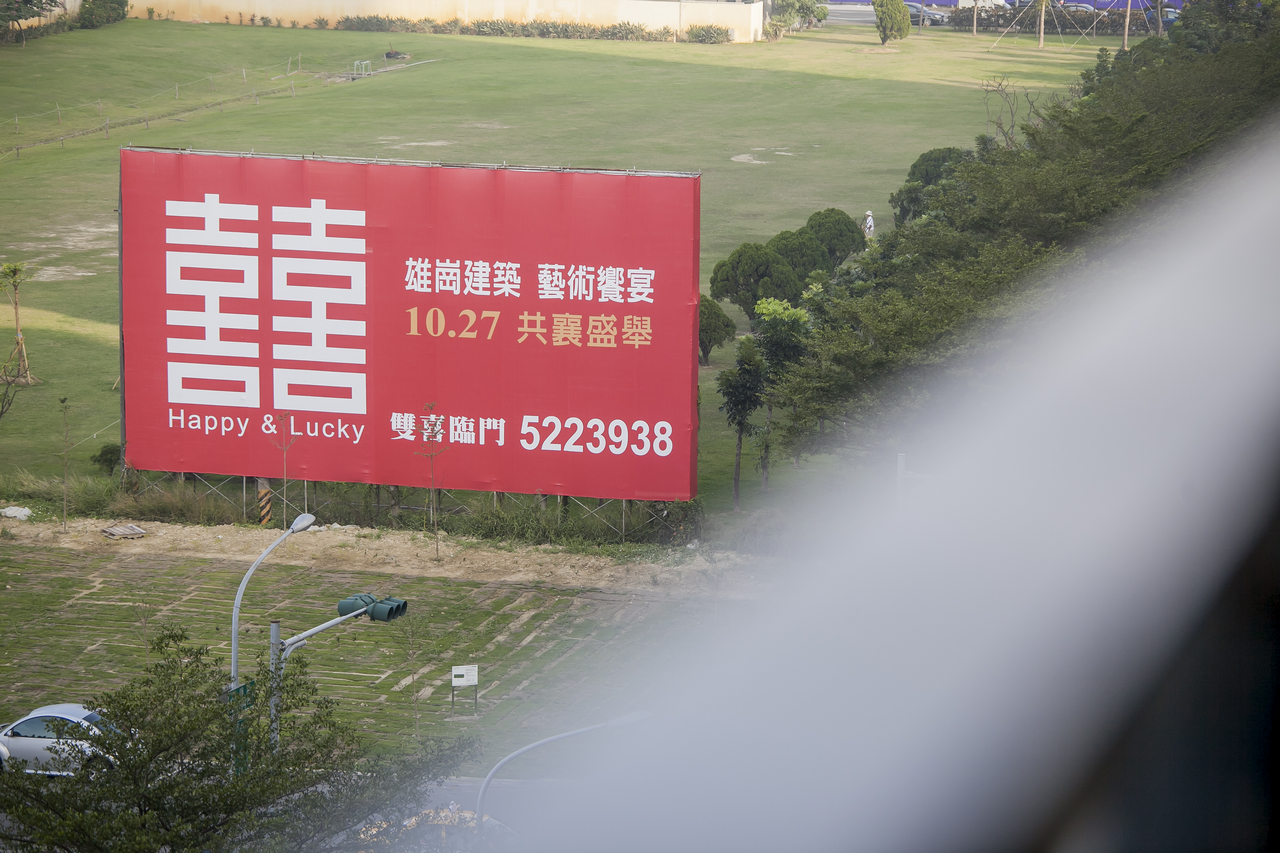The image features a prominent red billboard situated by the side of a road, set against a field of green grass with some bare patches. The billboard, adorned with a mix of Chinese characters and English text, prominently displays "happy and lucky" in white, flanked by additional Chinese characters. There is also a sequence of numbers, "5223938," and other text in yellow and white. The scene is framed by a tree line running along the road, with a few street lamps visible. Behind the trees, an individual dressed in white stands in a sprawling field. On the left side of the image, partially hidden by trees, a silver vehicle is parked. A blurry, white diagonal bar, possibly a part of a railing or barrier, stretches across the photo, suggesting the picture might have been taken from behind an obstructing object. Also visible is another street sign beside the road. The overall atmosphere is that of a clear daytime.